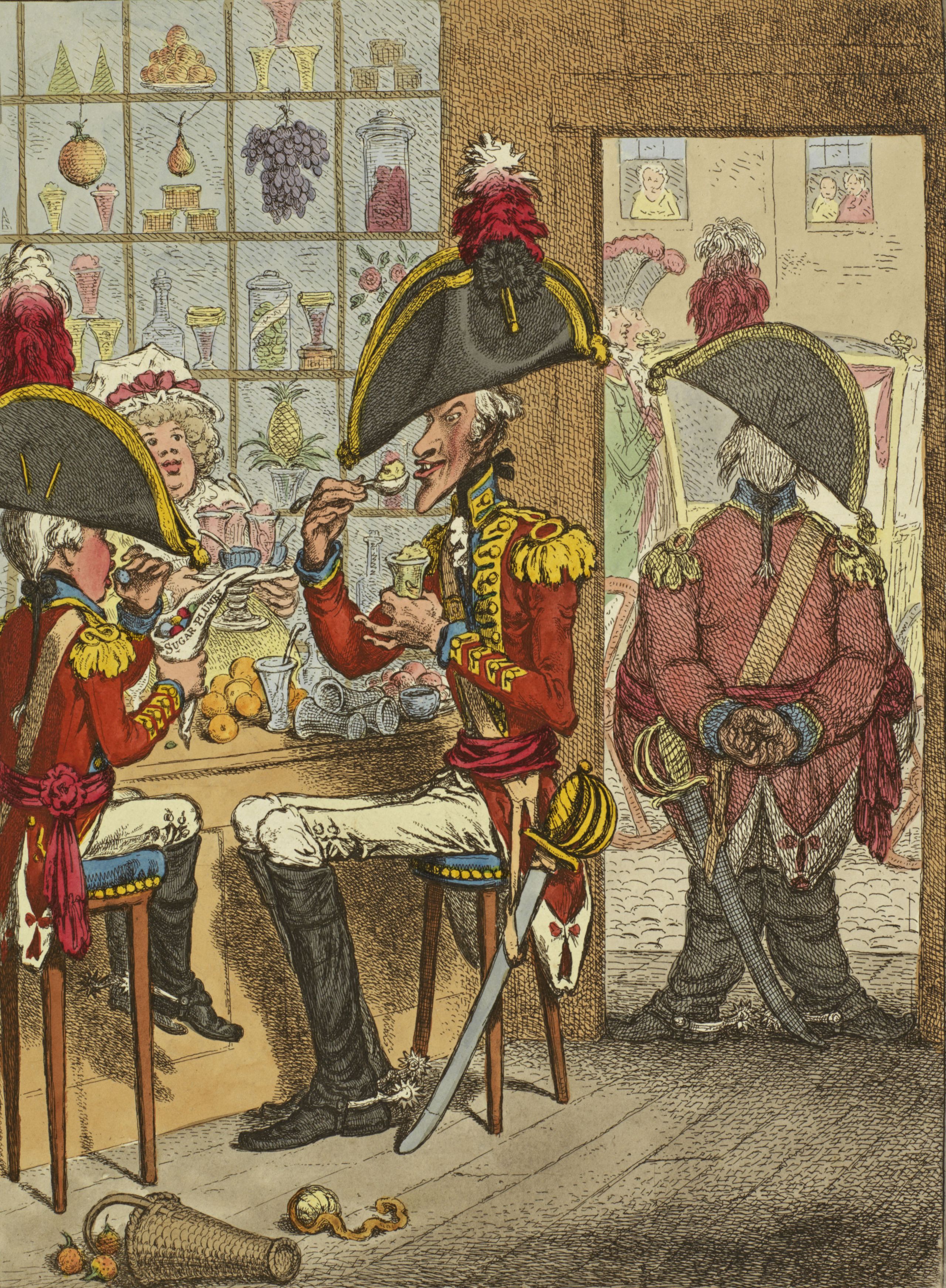This detailed illustration, possibly an antique-style cartoon or political comic, portrays a nostalgic bar scene featuring British soldiers. At the center, two soldiers in red coats with gold embellishments, tan pants, and black boots sit on wooden stools with light blue cushions, facing each other. One soldier's feet dangle from the barstool, mirroring the small boy beside him dressed identically, suggesting a whimsical or sentimental bond. The central soldier has a sheathed sword with a gold handle and a traditional black hat with gold trim sits on both soldiers, adding to their historical attire. They enjoy ice cream or food from a glass as they sit. 

Behind the bar, a woman looks on, surrounded by an assortment of items stored in wooden squares: bunches of grapes, cups, food, canisters, and a pineapple, further enhancing the setting’s rich detail. The left side of the floor displays a tipped woven basket with three orange fruits, possibly pomegranates, spilling out. Near the basket's edge lies a gold ornament with a long orange strip. 

On the right side, a soldier's back is to us, his hands clasped behind, possibly standing in front of a doorway that leads to another room suggested by a dusty brown background. This doorway hints at another engaging scene, perhaps a festive gathering. The upper left corner features windowpanes displaying various objects, anchoring the image in more elaborate detail. The light wood flooring transitions to a darker hue on the right, adding a sense of age and wear.